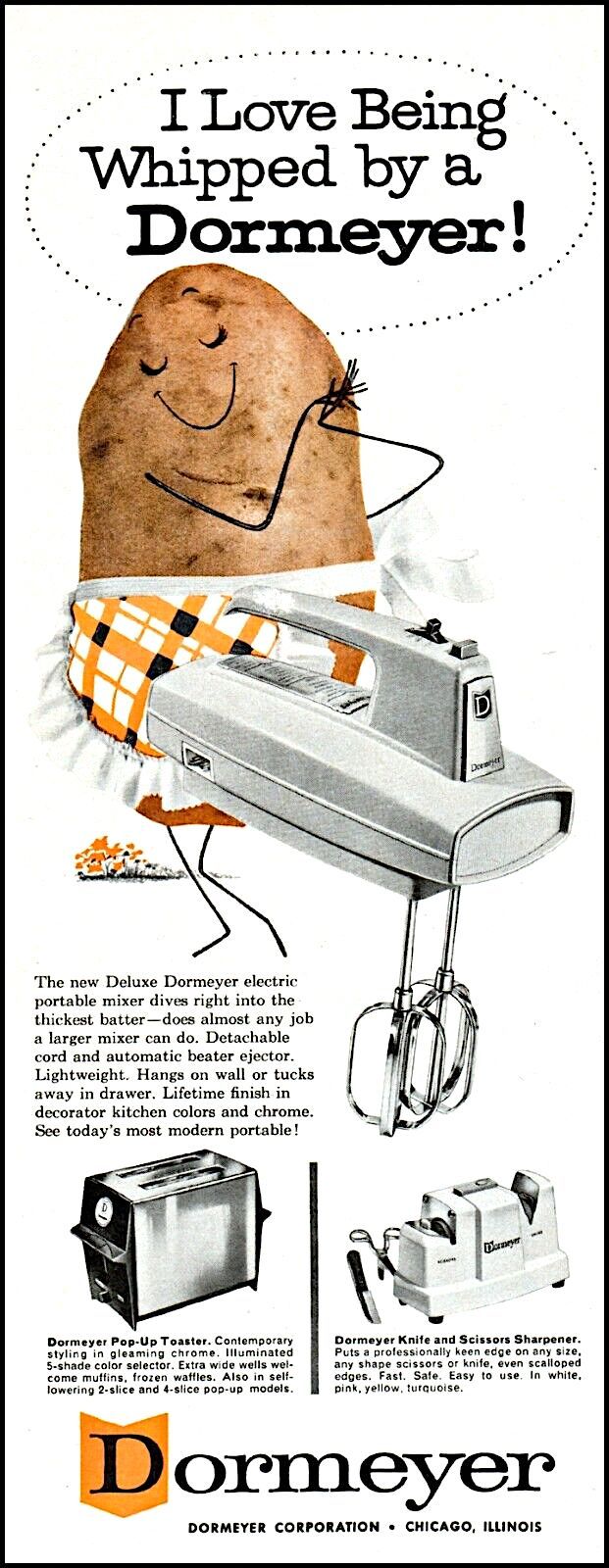The image is a vintage advertisement for Dormeyer appliances featuring a white electric portable mixer prominently displayed in the center. At the top of the ad, an eye-catching oval against a white background contains the bold black text, "I love being whipped by a Dormeyer." Beneath this, a whimsical potato character, wearing a gold apron with orange, black, and white stripes complete with ruffles, stands with its hands together, eyes closed, and a smile, conveying a sense of delight. The potato character humorously emphasizes the tagline. The mixer itself is illustrated with its beaters visible on the right side and a descriptive paragraph located below it on the left. To the left of the mixer’s description, the ad features a toaster, accompanied by its own description below it. To the right of the toaster appears a white knife and scissors sharpener. At the very bottom of the image, the advertisement is signed off with the name "Dormeyer" in an orange shield, followed by "Dormeyer Corporation, Chicago, Illinois."